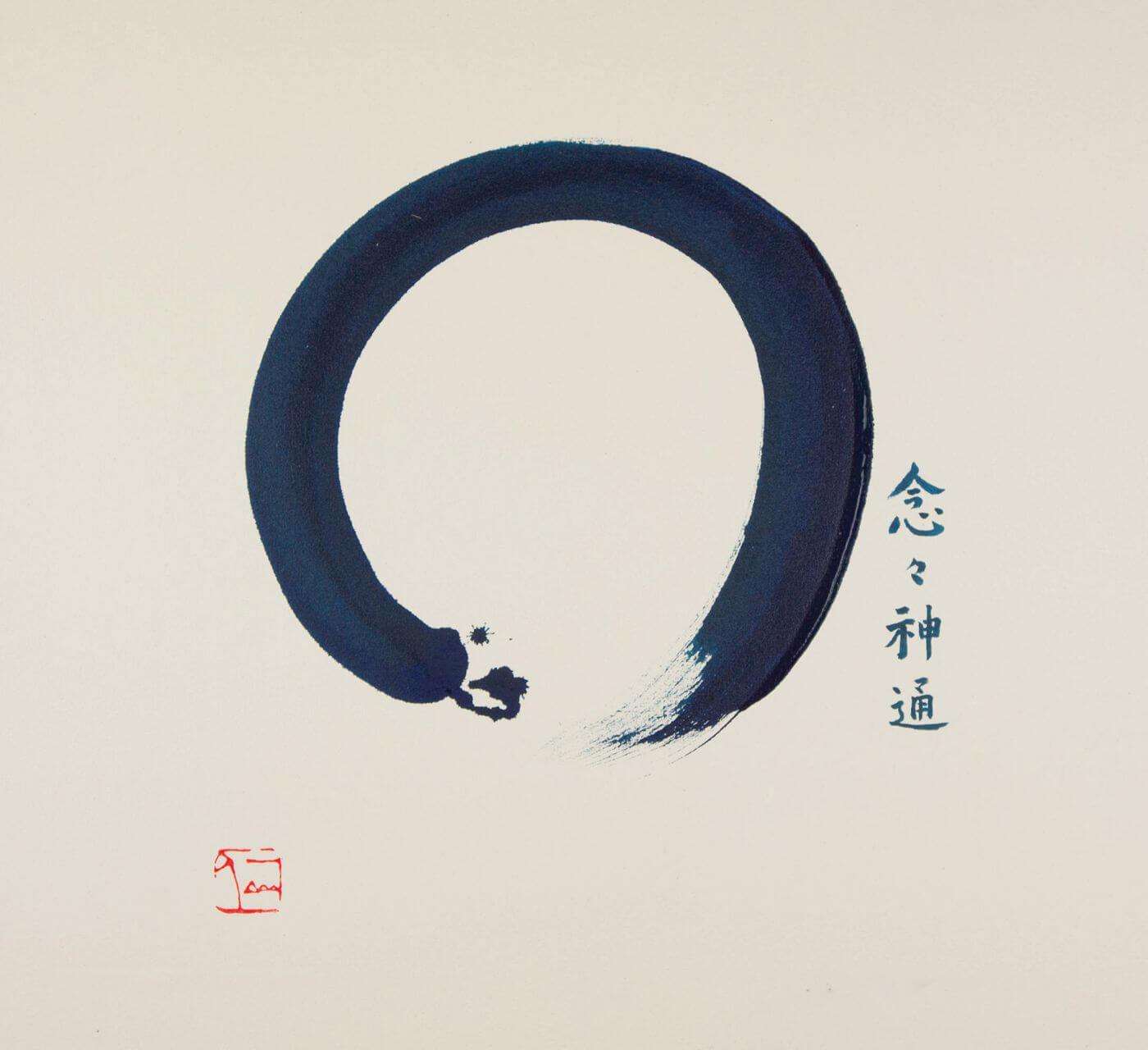The painting showcases a deep dark blue swirling circle on a cream-colored canvas background. The circle is almost complete, originating from the left side and curving around dynamically, leaving a trail of streaked paint as the brush lifts off the canvas before it can reconnect. This creates an impression of motion and energy. On the right side, four vertical Japanese symbols are elegantly rendered in a watery blue calligraphy. In the lower left-hand corner, a thin red symbol features a combination of lines and triangles, resembling an upside-down L and evoking a sense of intricate design. The composition harmonizes traditional and abstract elements, offering a visually captivating experience.